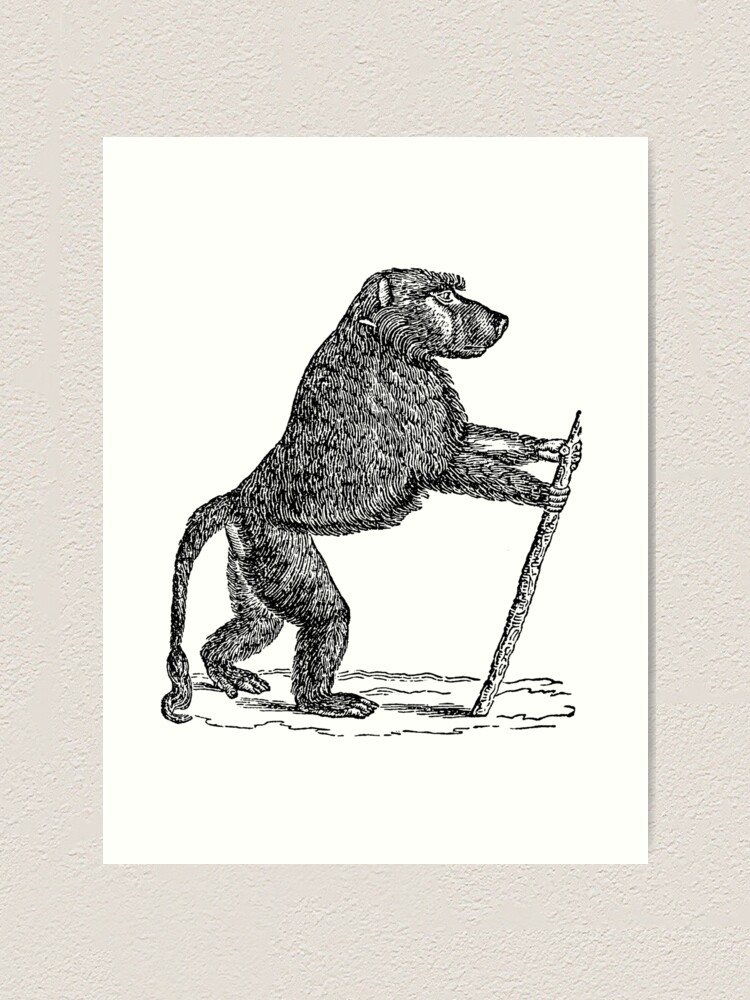A monochromatic illustration hangs on a pristine white stucco wall, drawn on a sizable sheet of white paper. The detailed black and white artwork depicts a monkey walking upright, holding a large stick akin to a walking stick. The monkey, with a notably long tail ending in a tuft of fur, appears to be gazing off towards the right side of the image. Beneath its feet, a series of squiggly lines suggest the texture of dirt, adding a sense of ground. The illustration skillfully incorporates shadows cast by both the stick and the monkey's feet, indicating that the scene is lit from the right, as if illuminated by the sun.